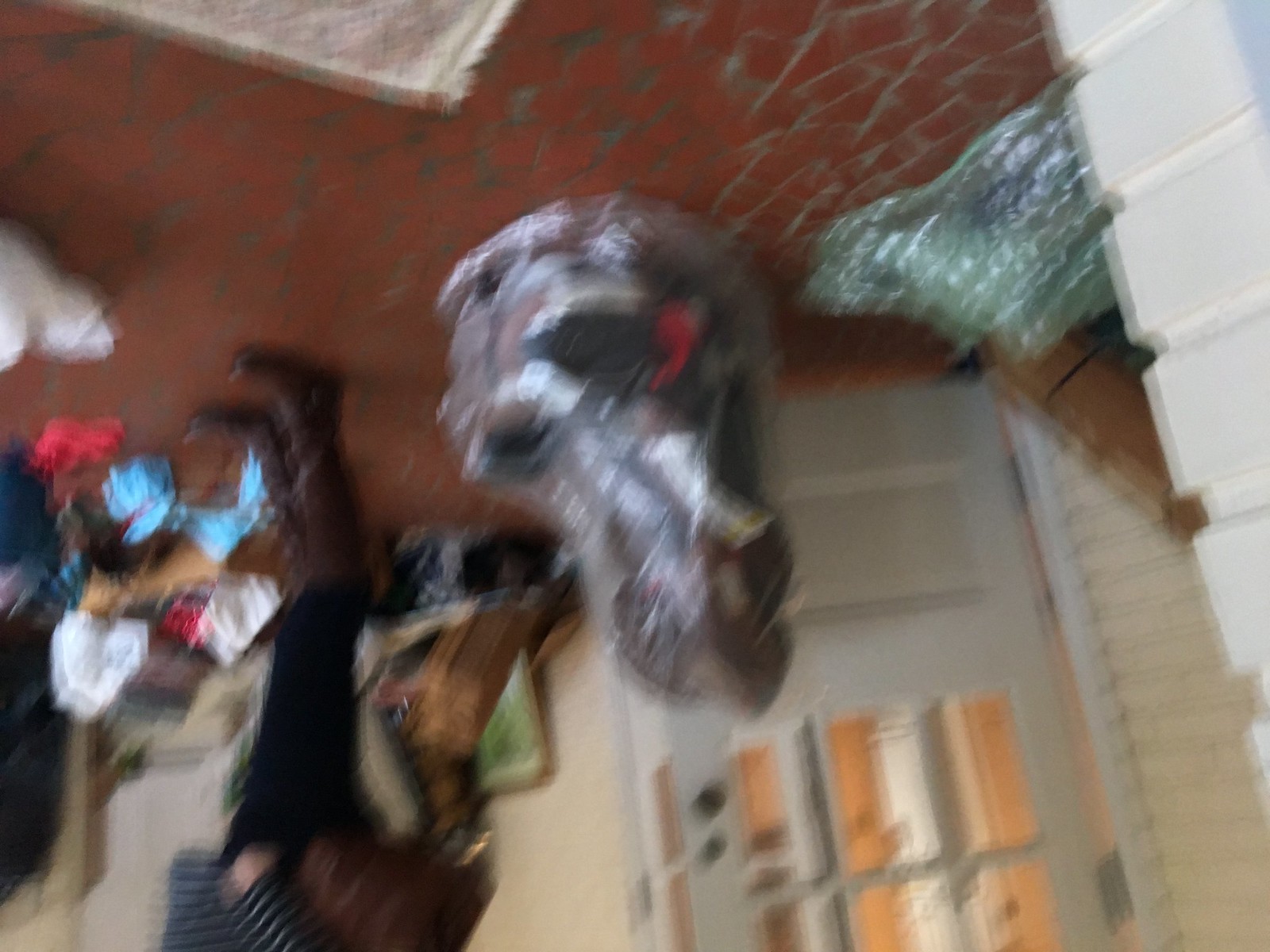The image is very blurry and appears to be taken upside down, causing an unusual perspective where the floor is located at the top. The floor, which is a shade of red, occupies the upper section of the photograph. Emerging from the top left-middle, there's a throw rug partially visible. On the actual top left side of the image, there's a white object that protrudes into view. At the center of the photograph, an item wrapped in cellophane is prominent, although its exact nature is indistinct due to the blurriness. To the left side of the image, a woman is partially visible; she is wearing boots and black pants but is cut off just above the waist, not showing her upper body.